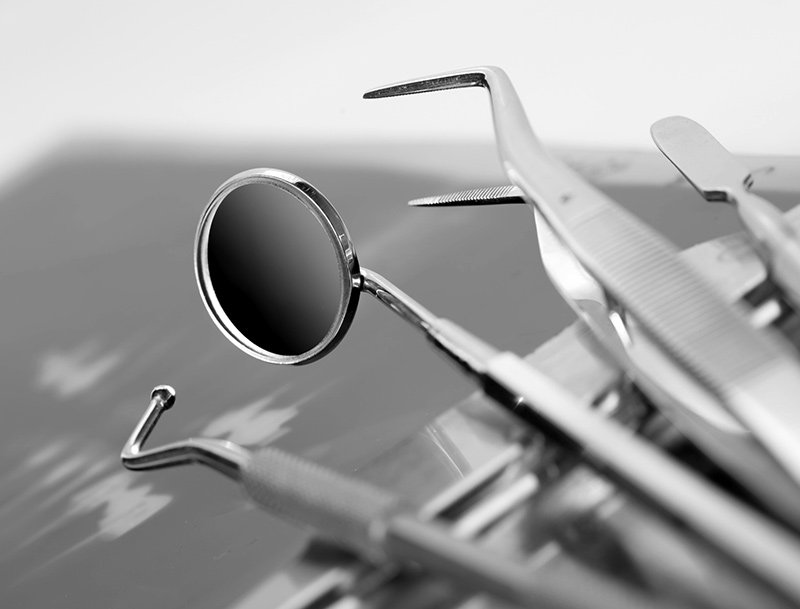The black-and-white image features a highly zoomed-in view of several dental instruments arrayed atop a stainless steel tray. Dominating the scene are various dental tools, including sharp picks, a hook-like tool with a ball end, tweezers, and a prominent instrument with a small dental mirror that partially reflects a gradient from black to gray. The instruments, all steel-colored and meticulously detailed, suggest a sterile, clinical setting. The background is nondescript and blurred, adding to the focus on the gleaming, clustered dental tools, making the image resemble a desktop wallpaper suited for medical or dental professionals.